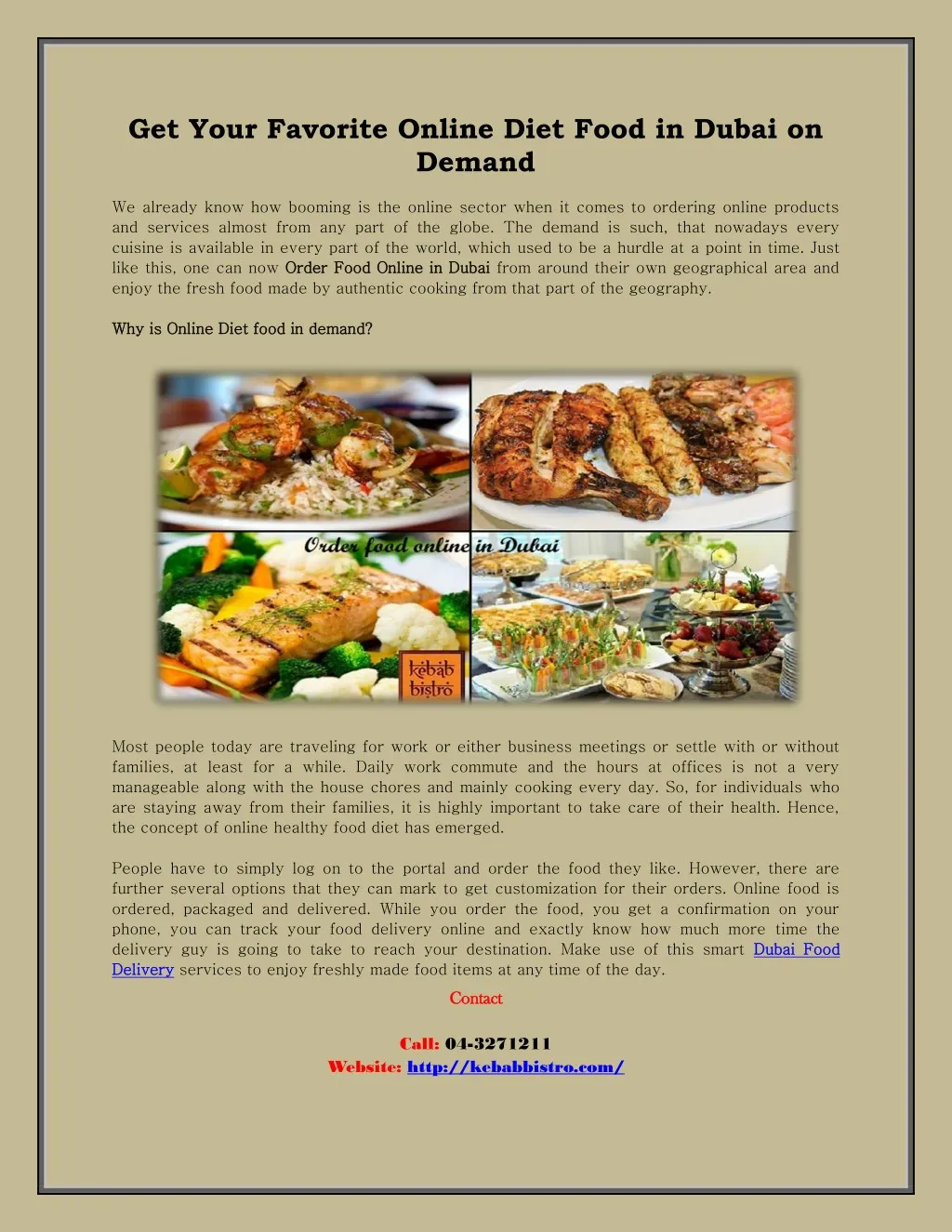The flyer features a title at the top in bold black type: "Get Your Favorite Online Diet Food in Dubai on Demand." Set against an olive green, almost beige background, the flyer is outlined with a black rectangle the size of a typical sheet of paper. Inside this outline, the flyer includes a range of textual and visual content. 

At the top, beneath the title, there's a paragraph that introduces the concept of booming online services and highlights the convenience of ordering diet food in Dubai from local sources. 

Slightly towards the top-middle section, there are four images showcasing diet food options, presumably available in Dubai. These images include dishes of chicken, cooked salmon, another piece of meat, and a spread of various foods. 

Following these images, further paragraphs delve into the reasons behind the popularity of online diet food services. It explains that many people, due to work or business commitments, are away from their families and find it challenging to manage daily meal preparations. 

The flyer concludes with a call-to-action, providing a phone number and a website at the very bottom for viewers to easily place their orders.